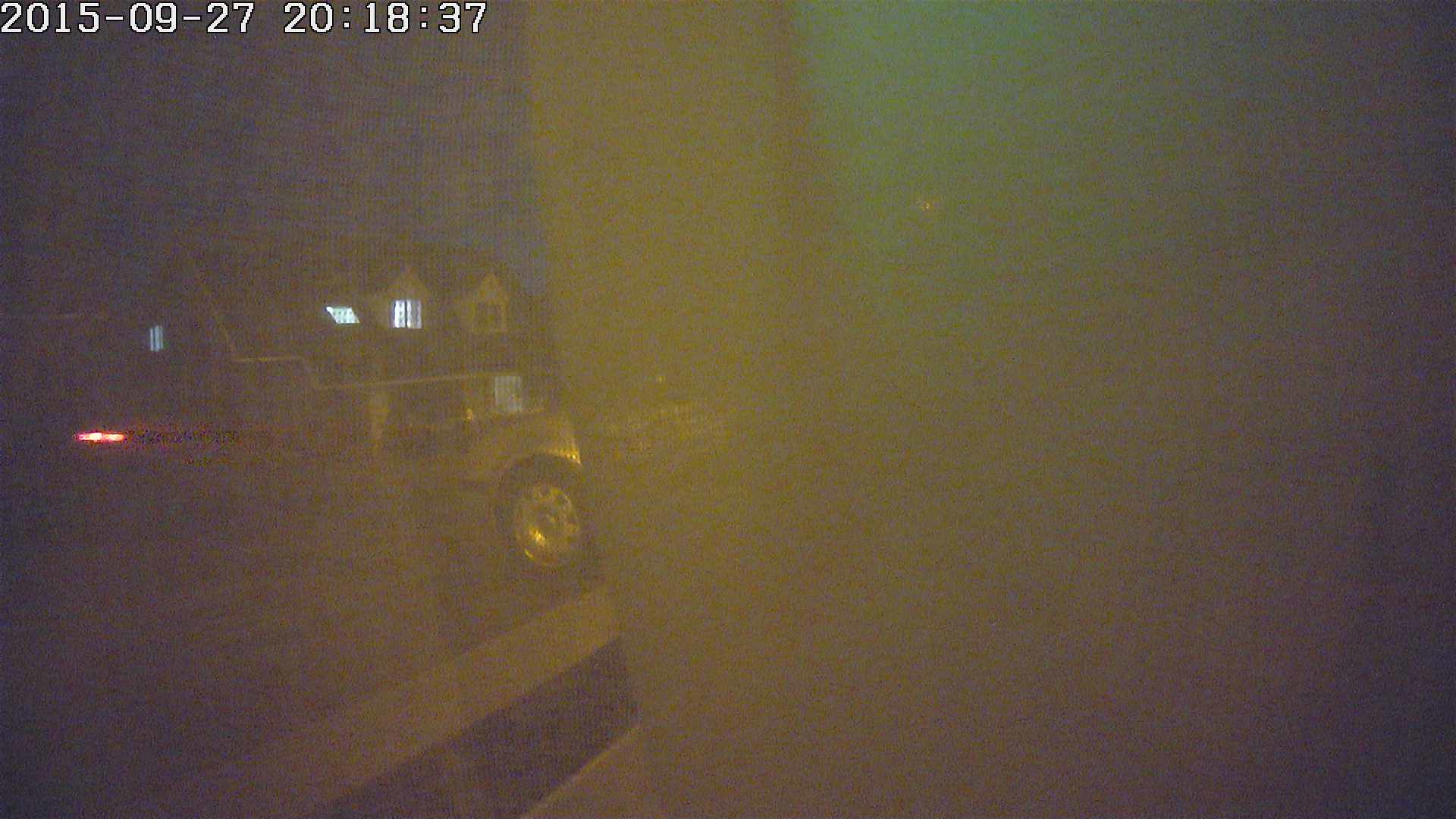The blurry nighttime image appears to be either security camera footage or taken through a window. Predominantly, it features a large white shape on the right side, which is darker at the right edge and lighter towards the left, possibly reflecting nearby lights. On the bottom left, a section of a white picket fence and the front fender of a silver car with a black wheel are visible. In the distance, there is a two-story white house with a dark roof, partially illuminated by lights from an attic window and other lower windows. Additionally, two red lights, likely from the rear of another vehicle, can be seen to the left of the photograph. This scene is timestamped in the top left corner with "2015-09-27 2018:37" in white text. The overall image is very dark, out of focus, and captured under low-light conditions, giving it a hazy appearance.